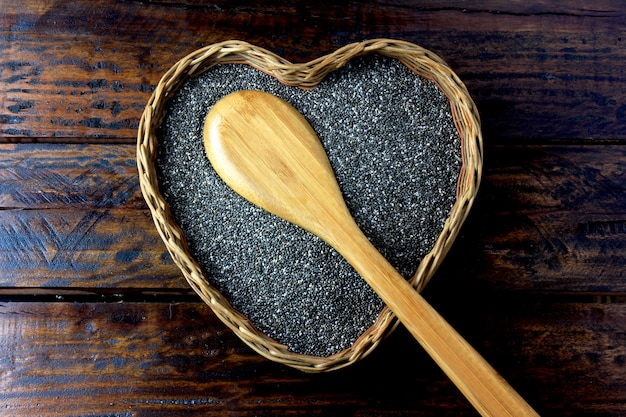This is a color photograph showcasing a rustic scene from a top-down perspective. At the center, there's a tan, woven wicker basket in the shape of a heart, sitting on a dark brown wooden table characterized by its visible grain and black grooves. The basket is filled with fine black grains, likely chia seeds or poppy seeds, creating a textured surface. Resting upside down on top of the grains is a large, light brown wooden spoon. The spoon's bowl is positioned in the top left corner of the basket, with the handle extending towards the bottom right of the image, partially disappearing out of the frame. The table and the objects are lit from the left, casting subtle shadows to the right, adding depth to the composition. The overall feel suggests a natural, home-crafted aesthetic, possibly reminiscent of a detailed product display seen on Pinterest.